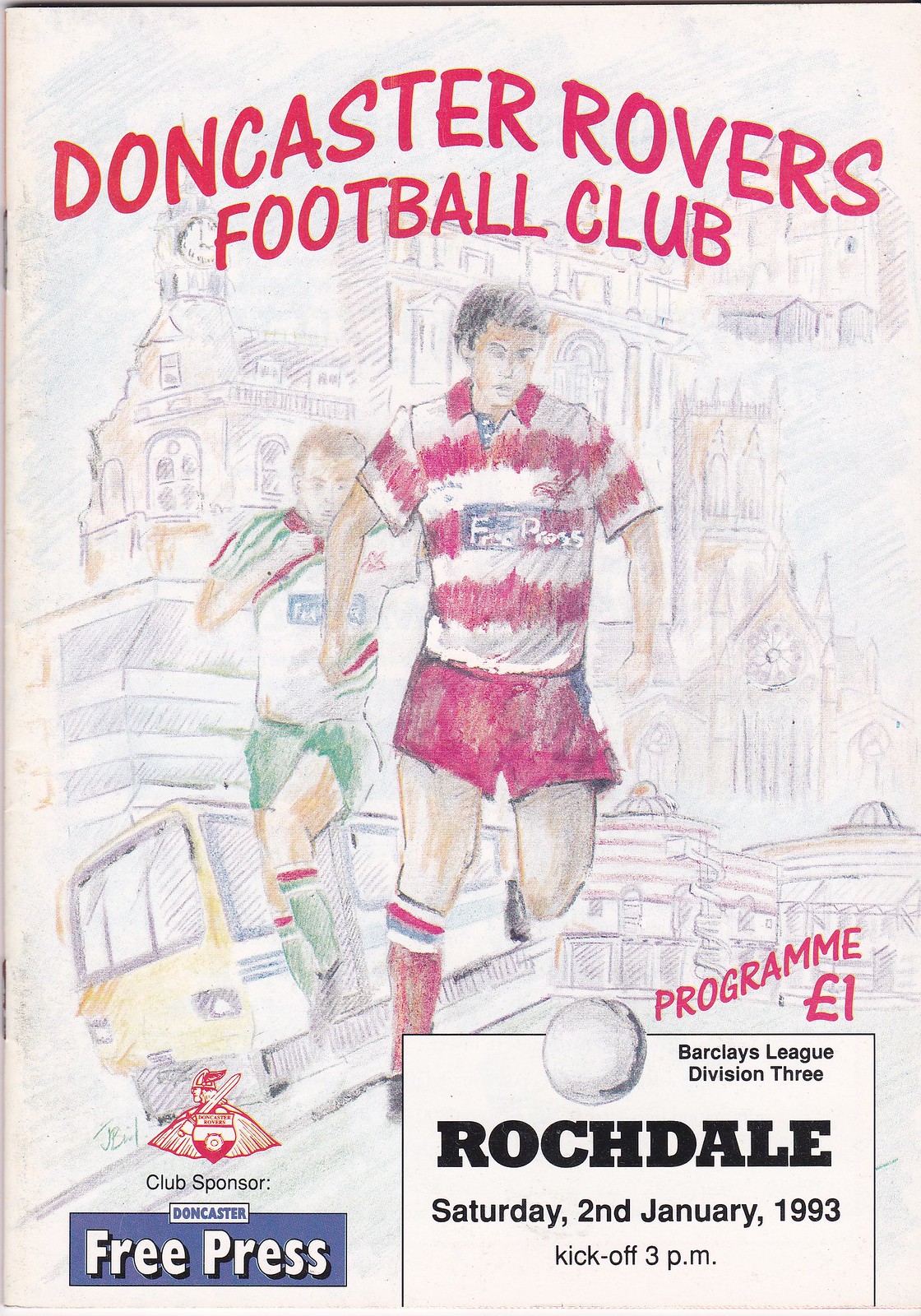This is a detailed image of a vintage soccer program cover, prominently featuring a sketched drawing that appears to be done with colored pencils or matte colors. Dominating the illustration are two soccer players: the main player is depicted in a red and white striped jersey with matching red shorts and socks, while the other player is in a blue, green, and white jersey with green shorts and socks, seemingly chasing the former with a soccer ball in play.

The background illustrates elements reminiscent of the UK, including buildings one might associate with Doncaster and a yellow train or bus, providing a distinct urban vibe. At the top, in bold red letters, the text reads "Doncaster Rovers Football Club." The cover is designed on a white piece of paper, enhancing the vintage feel.

In terms of textual elements, on the lower left corner, it mentions "Sponsored Club," and nearby, in a blue box, "Free Press," identifying the club's main sponsor. To the right, it displays "Program E1" in red, and beneath that, in black letters within a white box, the details read "Barclays League Division III. Rochdale. Saturday, 2nd January 1993. Kickoff at 3 pm," providing essential match information.